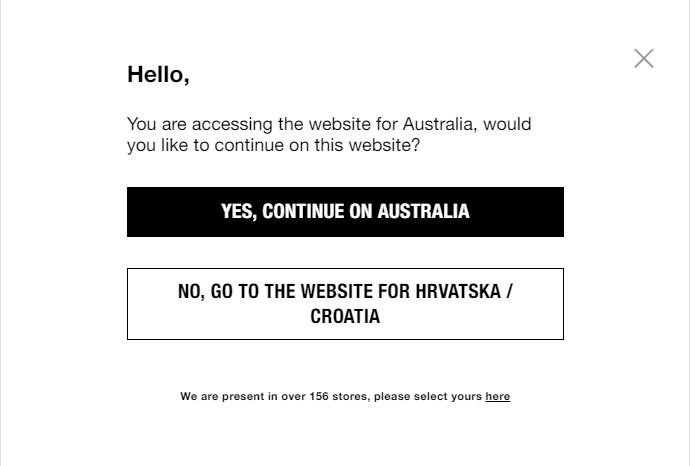The prompt on the website displays a message in bold text that reads, "Hello." The notice informs users that they are accessing the website intended for Australia and asks if they would like to continue with the Australian version. The option to proceed is presented in white text on a black bar, saying, "Yes, continue to Australia." Below this, there is another option in black text on a white bar that reads, "No, go to the website for Hrvatska (Croatia)." The mention of "Hrvatska" includes the spelling, H-R-V-A-T-S-K-A, for clarity. Additionally, there is information stating that the website is available in over 156 stores, and users are prompted to select their store by clicking an underlined link. In the upper right-hand corner of the message box, there is an X icon for users to close the prompt. The overall design is simple, aiming to direct users to the appropriate version of the website based on their location, a common feature on many international and retail websites to accommodate language and product availability variations.